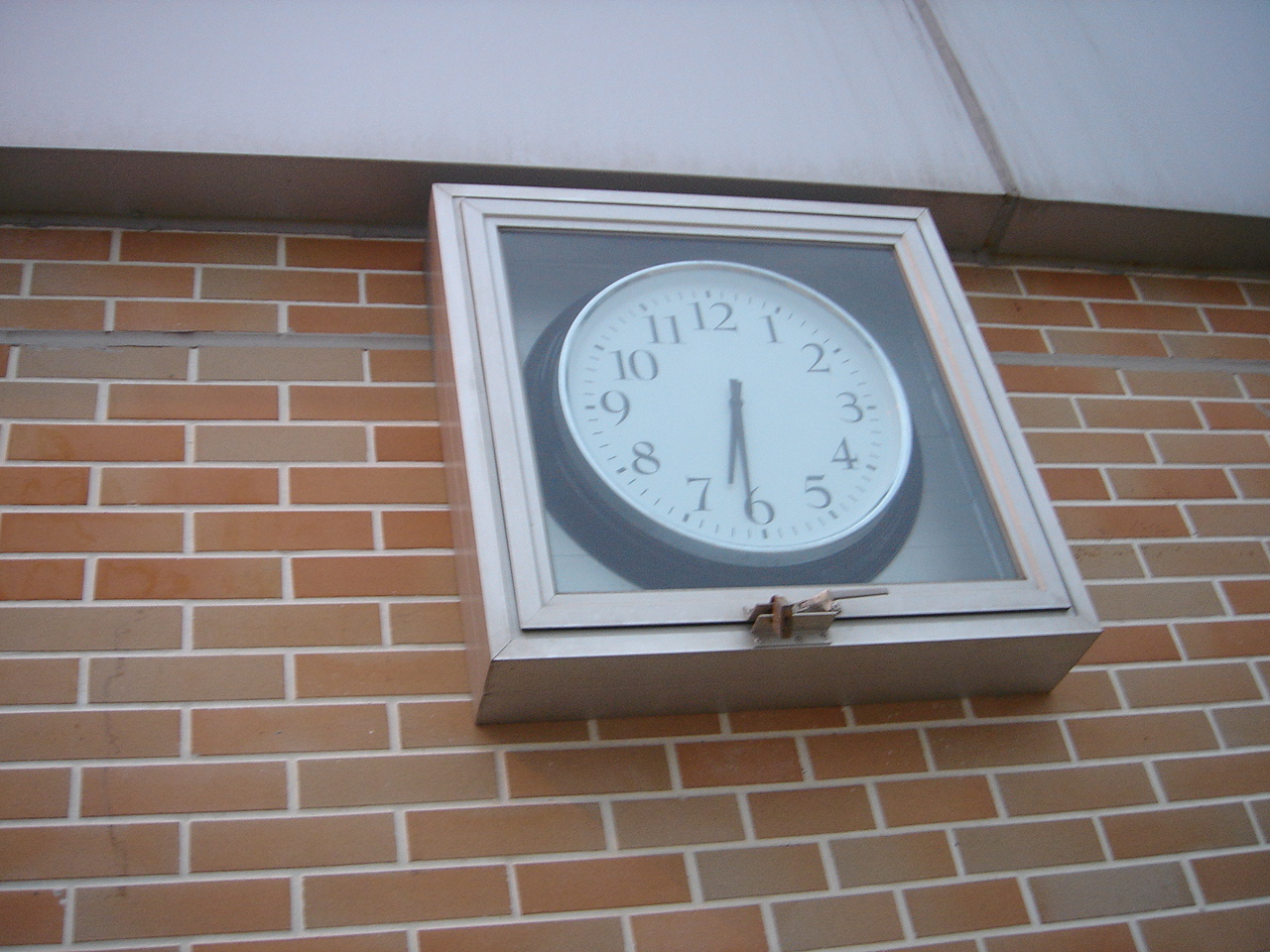The image showcases a black and white analog wall clock encased in a square, white or silver, transparent display case mounted on a brick-patterned wall. The clock, featuring a prominent black circular frame with a simple design, has black numbers from 1 to 12 and black hour and minute hands, but no second hand. The display case, which appears white or silver, is equipped with a hinge or latch for access. The wall behind the clock is reminiscent of a red brick school building, though it could alternatively be a brick-patterned design. A gray ledge, constructed from two large stone pieces, extends below the display case and matches the housing's width.